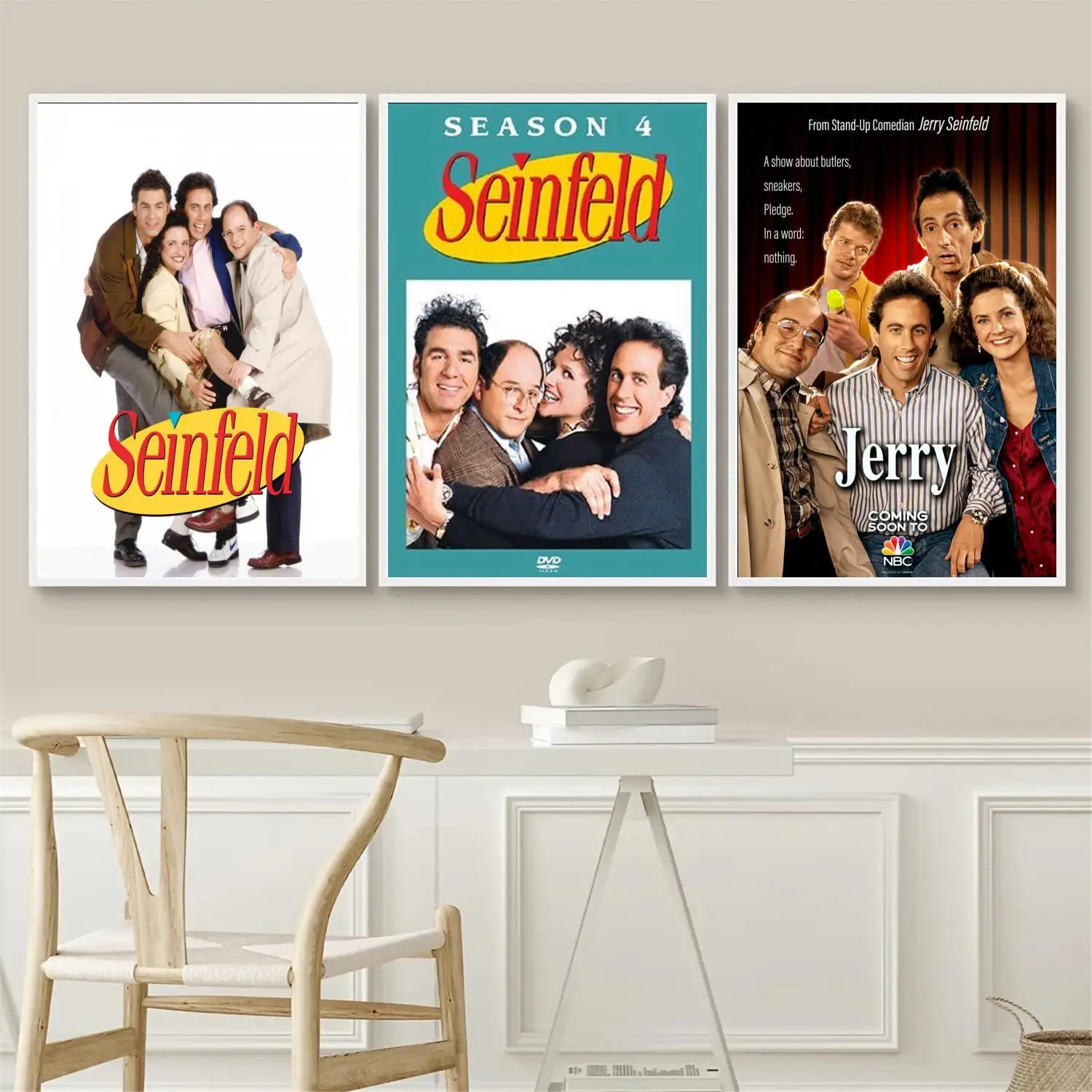The image depicts an interior scene with a detailed arrangement of Seinfeld-themed posters on a wall. The upper part of the wall has a light off-white paint while the lower third features bright white wooden paneling with raised Wainscoting. On the left, a light brown wooden chair with a white fabric seat is placed in front of the paneling. In the lower right corner, a portion of a woven basket is visible.

Three framed posters, each surrounded by a white border, dominate the wall. The first poster on the left showcases the cast of Seinfeld huddled together, set against a stark white background with a yellow oval at the bottom bearing the red Seinfeld logo. The middle poster is the DVD cover of Seinfeld’s Season 4, featuring a light greenish-blue background, white text at the top reading "Season 4," and a boxed image of the main characters huddled together with the word "DVD" in white text at the bottom. The rightmost poster focuses on the character Jerry Seinfeld, with the text "Jerry, coming soon to NBC" featuring the NBC peacock logo. The poster highlights a comedic premise about butlers, sneakers, and pledge with the famous tagline, "A show about nothing."

The arrangement and elements within the room emphasize a cozy domestic space adorned with prominent Seinfeld memorabilia.